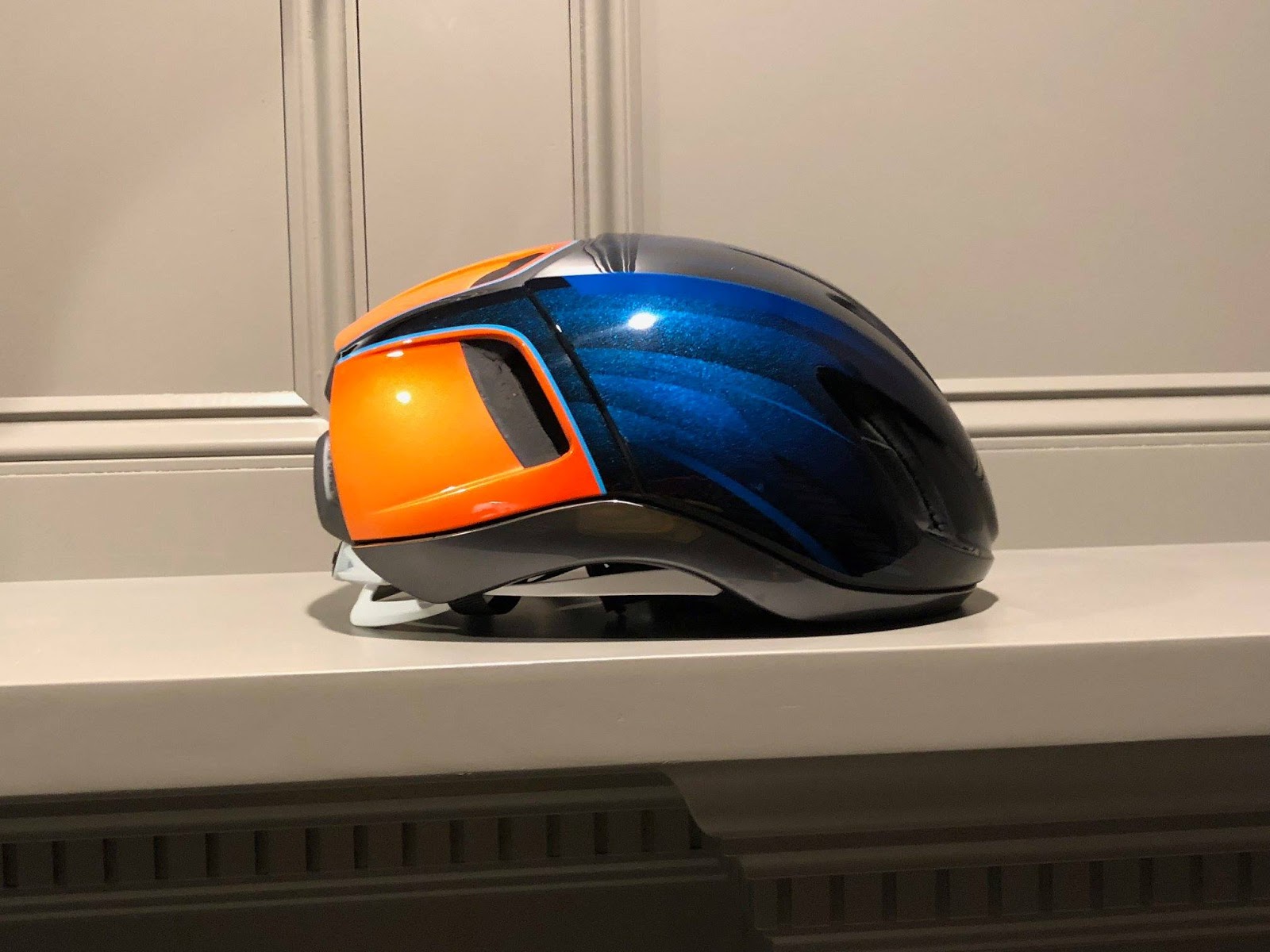The image is of a racing-style bicycle helmet prominently positioned in the center of the frame. The helmet features a striking, almost metallic, dark blue fluorescent color on the back half, seamlessly transitioning into vibrant orange details on the front. The helmet’s shell appears shiny and layered with varying shades of blue that glisten under direct lighting. An orange right-click and left-click button-like feature punctuates the design, along with a distinctive plastic white piece near the face portion. The background consists of a muted, cream-colored wall with wooden paneling beneath, painted similarly. The helmet rests on a narrow, tan or cream-colored shelf, aligned with part of a radiator visible below. The light casts a pronounced reflection on the blue section of the helmet, enhancing its glossy appearance. Colors in the frame include shades of blue, orange, black, gray, and silver, blending cohesively with the setting.